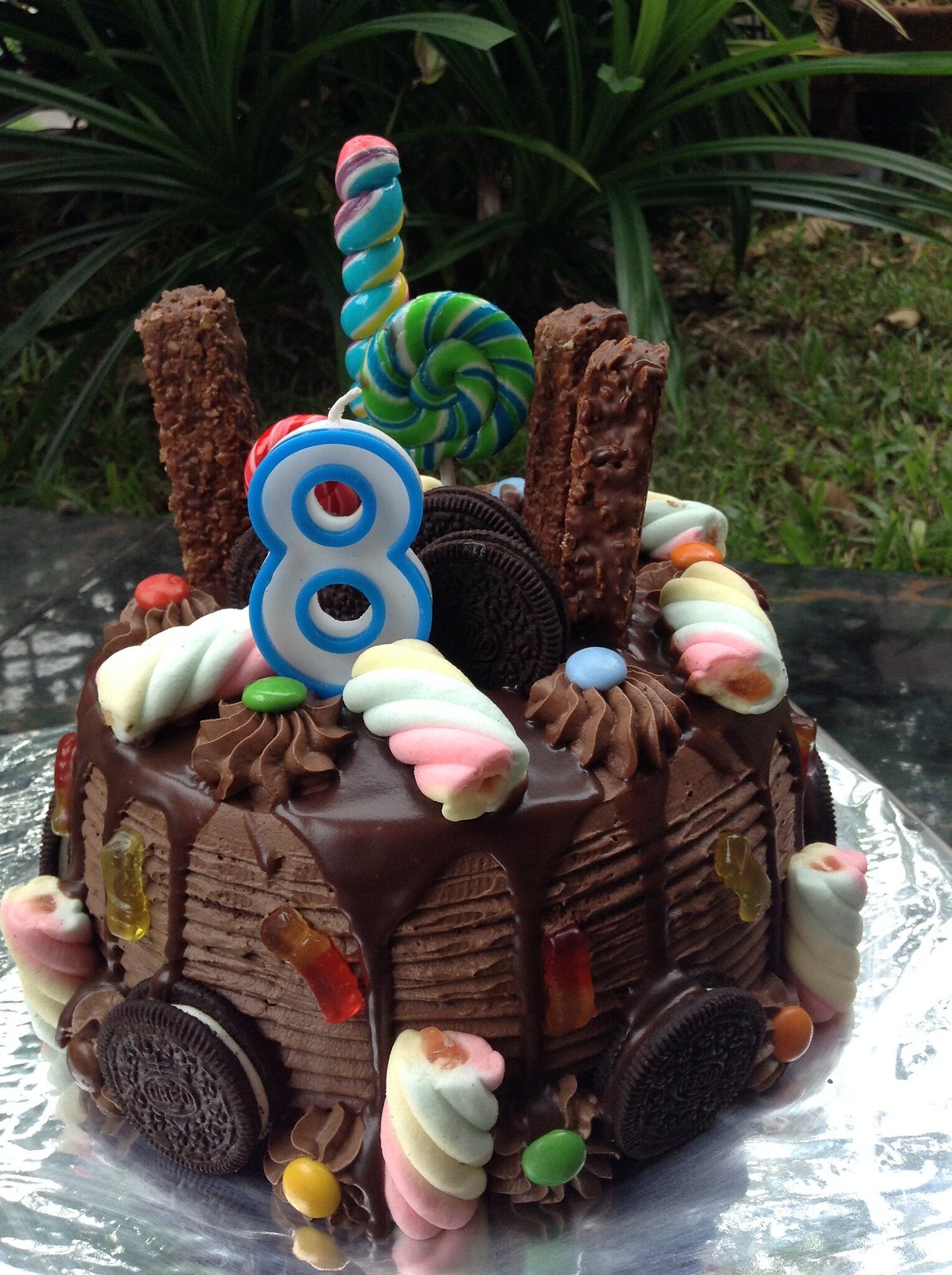The image showcases a lavishly decorated chocolate birthday cake, set outdoors on a piece of aluminum foil with a backdrop of grass and bushes. Centering the cake is a white candle outlined in blue, shaped like the number 8, indicating it’s for an eighth birthday celebration. The cake is enveloped in chocolate frosting, with a thick, dark fudge sauce artistically dripping down its sides in a comb effect. Adorning the cake are an array of delectable decorations: rosettes in lighter dark chocolate topped with colorful M&Ms, Oreo cookies embedded both on the sides and top, and intricate marshmallow twists in hues of pink, yellow, and blue. Additionally, gummy worms, or bugs, crawl along the cake, adding a playful touch. Among the embellishments on top, there are two upright chocolate wafers, a twisted blue, yellow, white, and green lollipop, and another round swirl lollipop, creating a vibrant and festive appearance. This meticulously decorated cake is clearly the centerpiece of an outdoor celebration, exuding creativity and charm against the natural scenery.